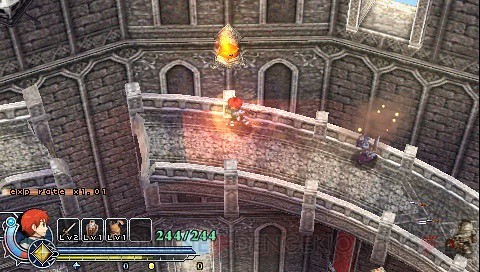In a vivid scene reminiscent of a fantasy video game, the image showcases a grand, circular stone tower, or perhaps a castle, constructed from gray stone. A mystical ambiance is enhanced by the warm glow of at least one torch mounted on the wall, casting flickering flames. Central to the image, a human-like character with striking red hair clad in light-colored garments stands on a crumbling spiral bridge that ascends the tower. This character faces left, towards a missing segment of the bridge they are approaching, engulfed in a radiant orange aura, possibly flames.

Trailing behind the red-haired figure is another character, distinguishable by their darker, blue and purple appearance, also shrouded in a faint yellow haze, contributing to the scene’s ethereal atmosphere. The entire setting appears to be within a large, circular stone chamber, with the bridge spiraling upward in an almost enchanting manner.

In the lower left corner of the image, there is a character interface displaying important information. This interface includes various boxes and icons, such as swords and other objects, indicative of the character's inventory or abilities. Prominent within this informational area are a blue bar and a yellow bar, likely representing the character's health and mana or stamina. An icon depicting the red-haired character provides a quick-reference visual, accompanied by more detailed character stats and information.

Overall, the visual encapsulates the essence of a medieval fantasy adventure, drawing viewers into its captivating world through detailed artistic elements and immersive character dynamics.